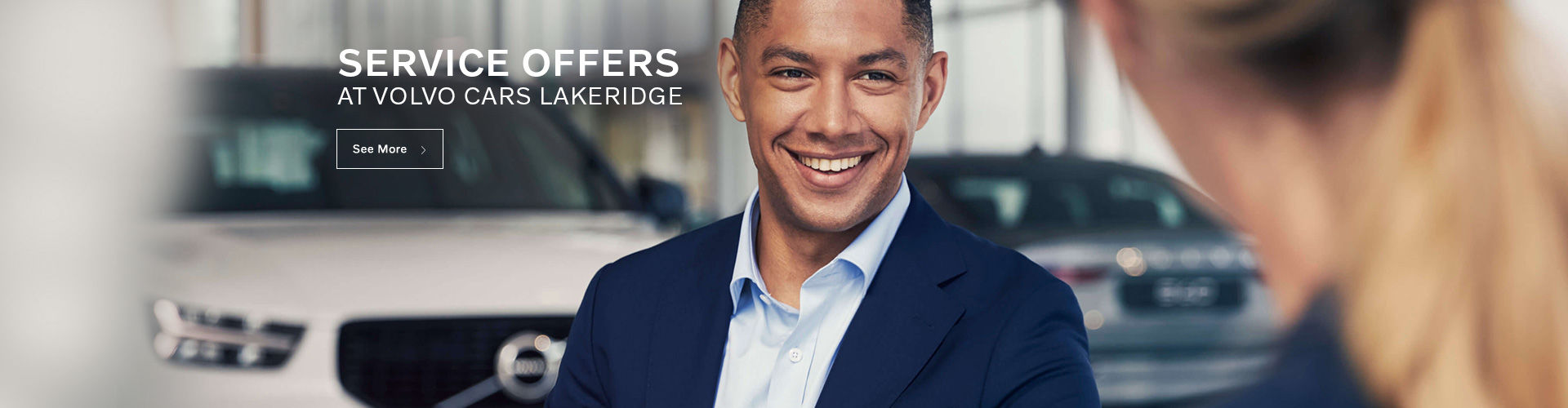A well-dressed gentleman, presumably of African descent, stands smiling in the center of a car dealership showroom. He is attired in a blue blazer over a light blue shirt with the top button undone, exuding a friendly and approachable demeanor. Behind him, a white Volvo sedan faces towards him, with the recognizable Volvo emblem featuring a diagonal bar subtly visible. Over his left shoulder, a silver, possibly bluish-colored car, also appears to be a Volvo, albeit blurrier as it is positioned further back. On his right, a woman with blonde hair tied up in a ponytail, dressed in business attire, can be seen, although she is somewhat obscured and blurry. Both individuals seem engrossed in what appears to be a polite, possibly professional conversation, contributing to an atmosphere of amiable interaction and professionalism in the car dealership setting.